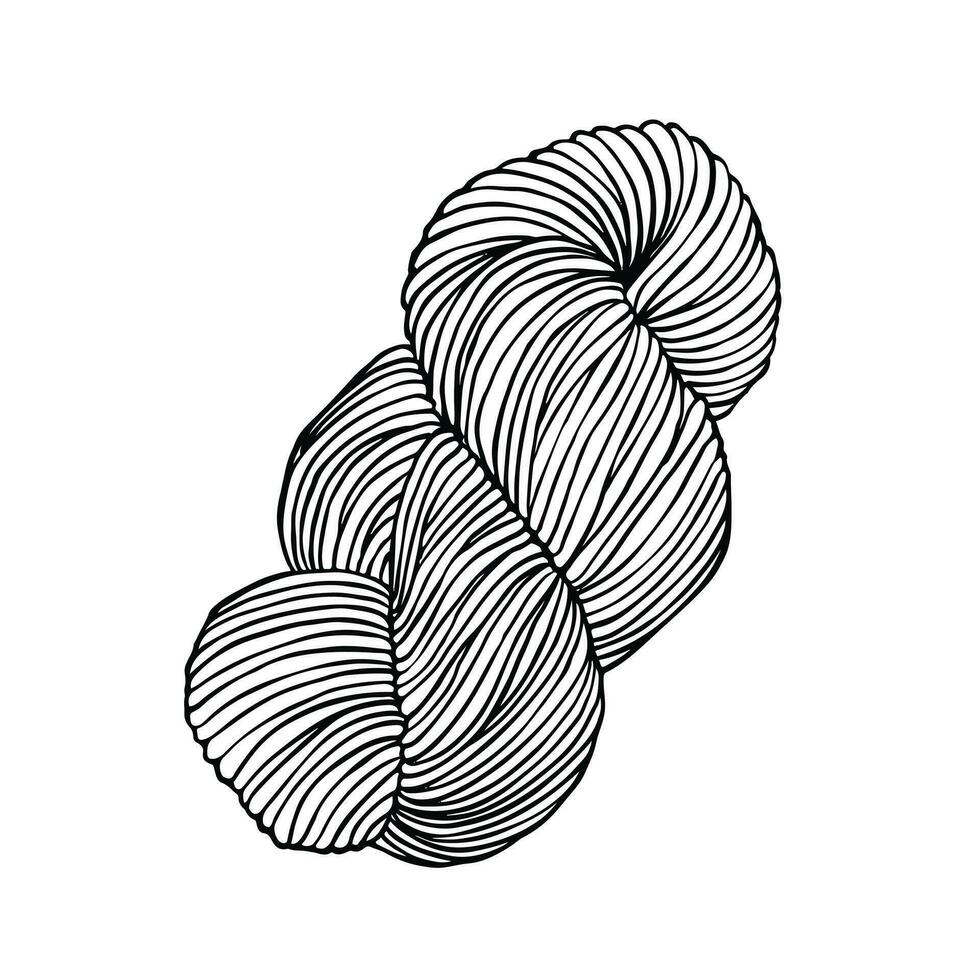This image features a detailed black and white pen-and-ink drawing of a skein of yarn, set against a flat white background. The skein of yarn curls and twists intricately around itself, with individual strands clearly visible. The smooth edges and the detailed line work give it a refined appearance. The skein is positioned diagonally from the lower left to the upper right, creating a dynamic orientation. This minimalist depiction captures the texture and form of the yarn, reminiscent of modern art interpretations or even the swirling lines of a slinky or twisted pastry bread, illustrating the endless possibilities of the subject matter in its abstract form.